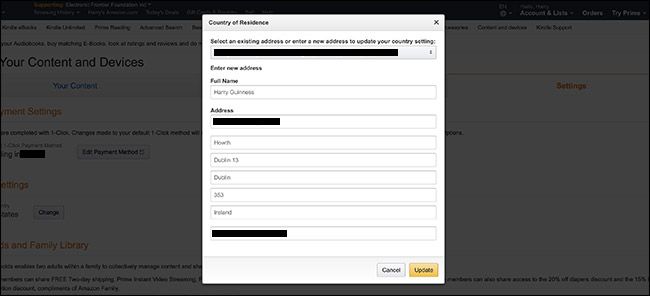The image depicts a computer screen showing a webpage titled "Your Content and Devices." A pop-up rectangle overlay within the page is prominently displayed in the foreground. At the top of this pop-up, the bold title "Country of Residence" is visible, accompanied by instructions to “select an existing address or enter a new address to update your country setting.” 

The user's privacy measures are evident as black rectangles have been strategically placed to obscure sensitive information. One such black rectangle hides the currently entered address. Below the instructions, there's a partially visible name, "Harry Guinness," and the street address, too, has been concealed with a black rectangle.

Additional elements on the pop-up include the mention of "365 friends," a country label that says "Ireland," and further privacy-protected information indicated by another black rectangle. At the bottom of the pop-up, there are two actionable buttons: a grey "Cancel" button on the left and a highlighted yellow "Update" button on the right.